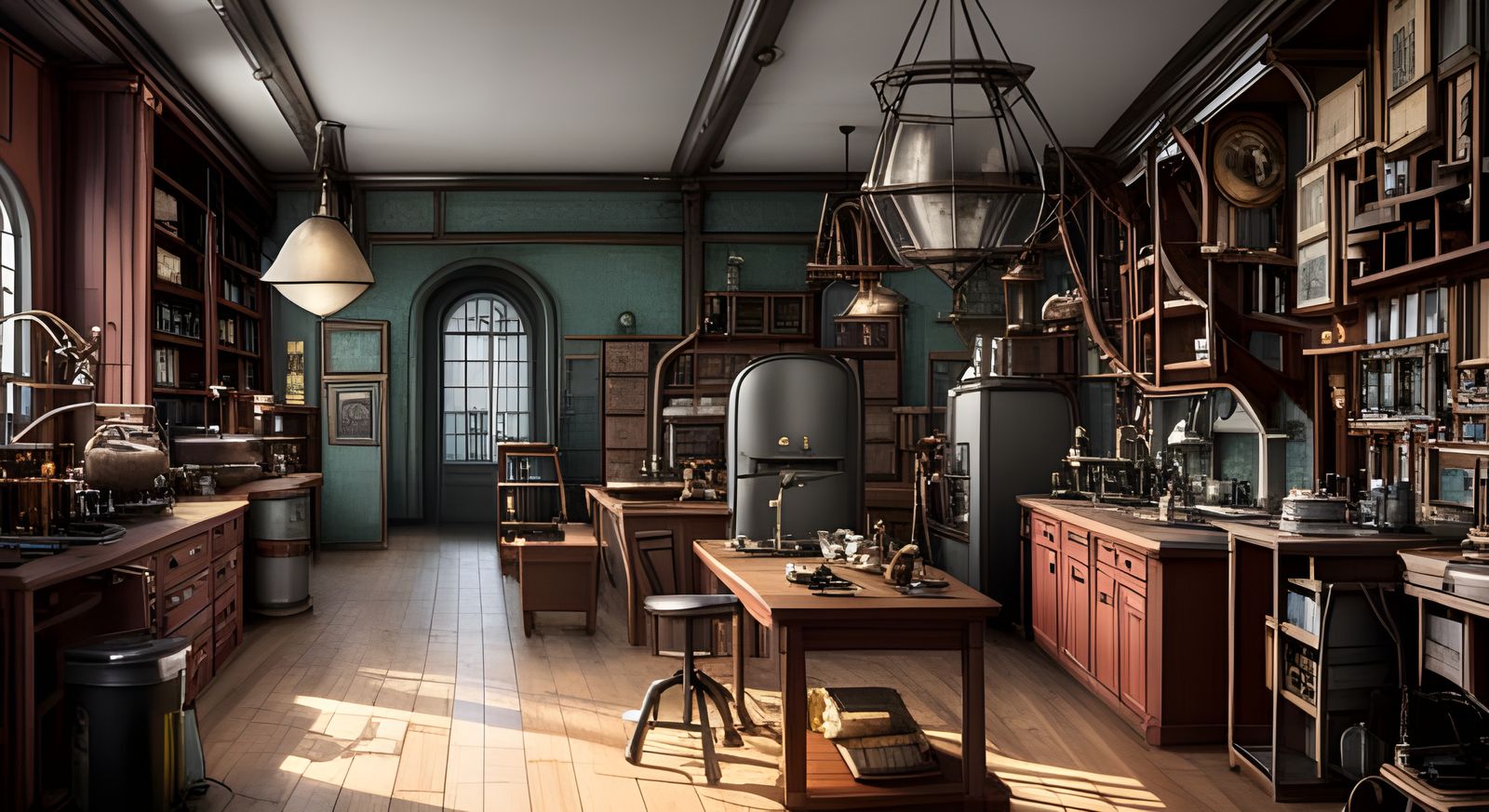The image depicts a highly detailed digital art painting of a vintage laboratory room with a realistic touch. The room features a light brown wooden floor and a sturdy, brown wooden table situated at its center, adorned with various scientific instruments and apparatus. Adjacent to the table stands a four-legged stool with wheels and a round, rotating top. 

The walls on either side of the room are lined with cabinets, drawers, and open shelves filled with assorted scientific equipment, including pots on long arms and silver metal apparatuses, evoking an aura of an early era scientist's workspace. The right wall is decorated with paintings, adding to the room's intellectual ambiance. 

The room is illuminated by multiple lights hanging from a white ceiling supported by black structural elements. Natural light filters in through a window on the left wall, casting sunbeams onto the floor, while the bluish front wall features a large, multi-paned arched window opposite the scene. A refrigerator can be seen along the back wall, further hinting at the laboratory's vintage setup. Additionally, there is another large refrigerator-like structure in sight, enhancing the sense of a well-equipped yet historical scientific environment. A large, round garbage can sits in the bottom left, completing this meticulously organized and evocative scene.